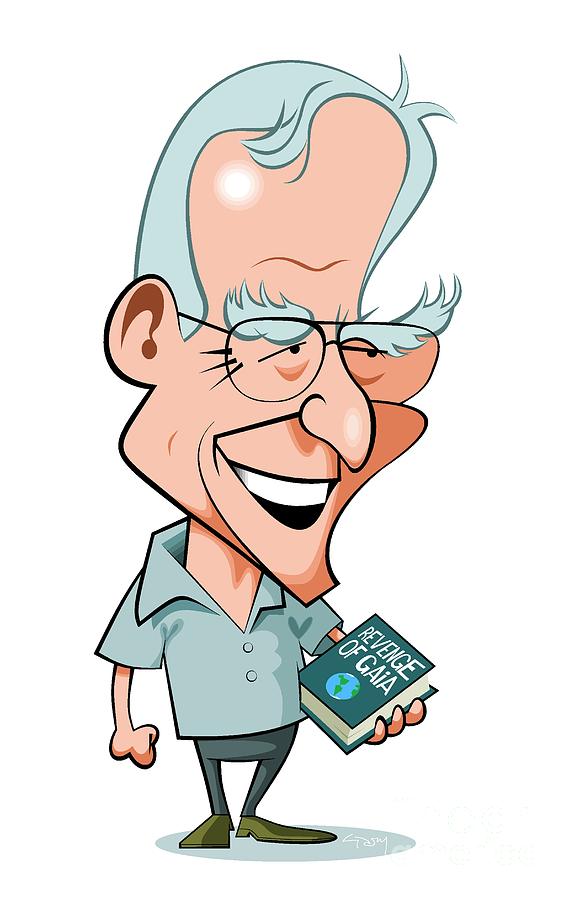This illustration is a caricature of an elderly man with exaggerated features, most notably a disproportionately large head compared to his small body. His large, bushy gray eyebrows match his short gray hair, and he sports a pair of glasses. The man's expansive forehead adds to the comedic effect of the caricature. He wears a light blue short-sleeved collared shirt, dark gray pants, and brownish-tan shoes. His expression is jovial, displaying a broad smile with his teeth showing. One hand holds a book titled "Revenge of Gaia," which is dark blue and features an illustrated globe with green continents, particularly North and South America, on its cover. His other hand is positioned downwards, making a fist. The overall portrayal is humorous and vivid, emphasizing the man's cheerful demeanor and the prominent size of his head.